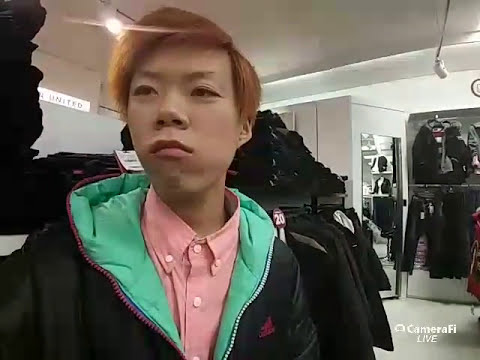The image depicts a young Asian male or older teen boy standing in a clothing store. The store’s interior features white walls, floors, and ceiling, with various clothes arranged on racks to both sides. The right side also has clothes hung on the wall alongside a mirror. The boy stands slightly to the left of the image, wearing a fashionable outfit that includes a black jacket with a light aqua green inner lining and a pink button-down shirt underneath. Notably, his jacket has red and white zippers, and he has medium-length orange hair. He appears to be looking away from the camera, potentially trying on clothes, and has a somewhat disappointed or upset expression. In the lower right corner of the image, text reads "Cameraify Live" in small white letters.